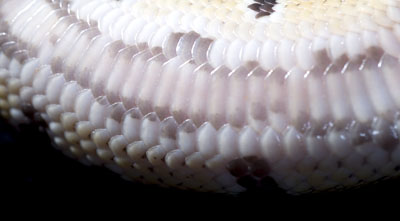This detailed image captures an extremely close-up view of a snake's skin. The background is entirely black, providing strong contrast. The prominent focal point is the intricate patterns of the snake's scales. The scales vary in shape, appearing as a mix of small rectangles, squares, and circles, resembling tiny corn pellets. Predominantly white, the scales also exhibit shades of tan, light gray, brown, and yellow, with intermittent red stripes adding visual interest. The various colors create a fascinating, albeit non-uniform, mosaic. Despite not showing the snake's head, tail, or entire body, the precision and detail of the scales are highlighted. The bottom part of the image is darker, drawing attention upward to the textured snake skin.